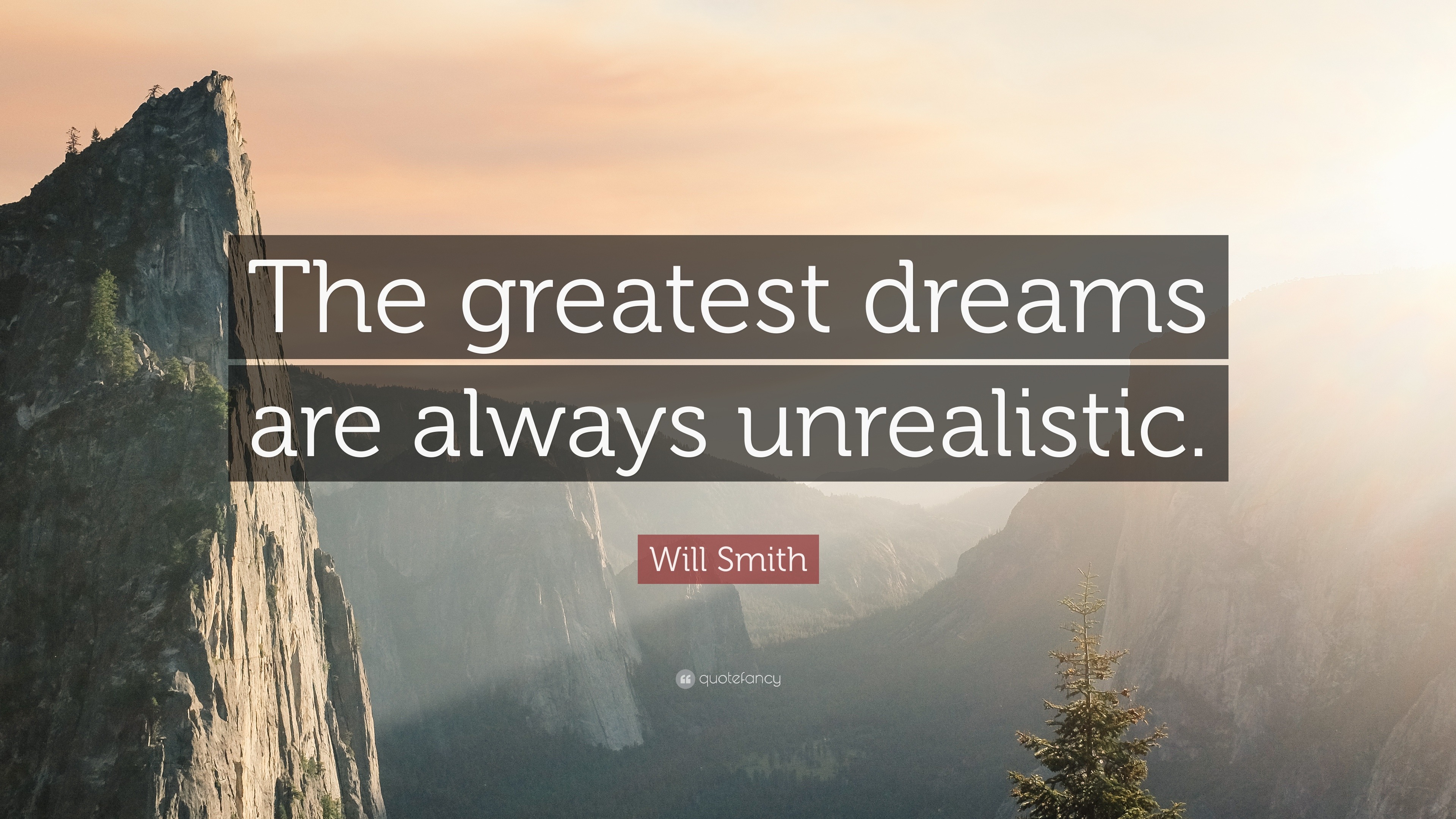The image is a striking motivational poster featuring a breathtaking view of high cliffs or canyons in a majestic valley. The rocky mountainous region is adorned with hardy green trees scattered across the surfaces of the cliffs. The sun peeks over the right side of the photograph, casting its rays to illuminate the entire scene. In the lower right corner, the top of a pine tree is visible. 

Across this inspiring natural backdrop, the quote "The greatest dreams are always unrealistic" is displayed prominently in white font, with a faint translucent black border around the text for emphasis. Below the quote, the name "Will Smith" is highlighted in white text with a translucent red border. The poster appears to be sourced from a site called Quote Fancy, as indicated by the smaller text beneath the quote.